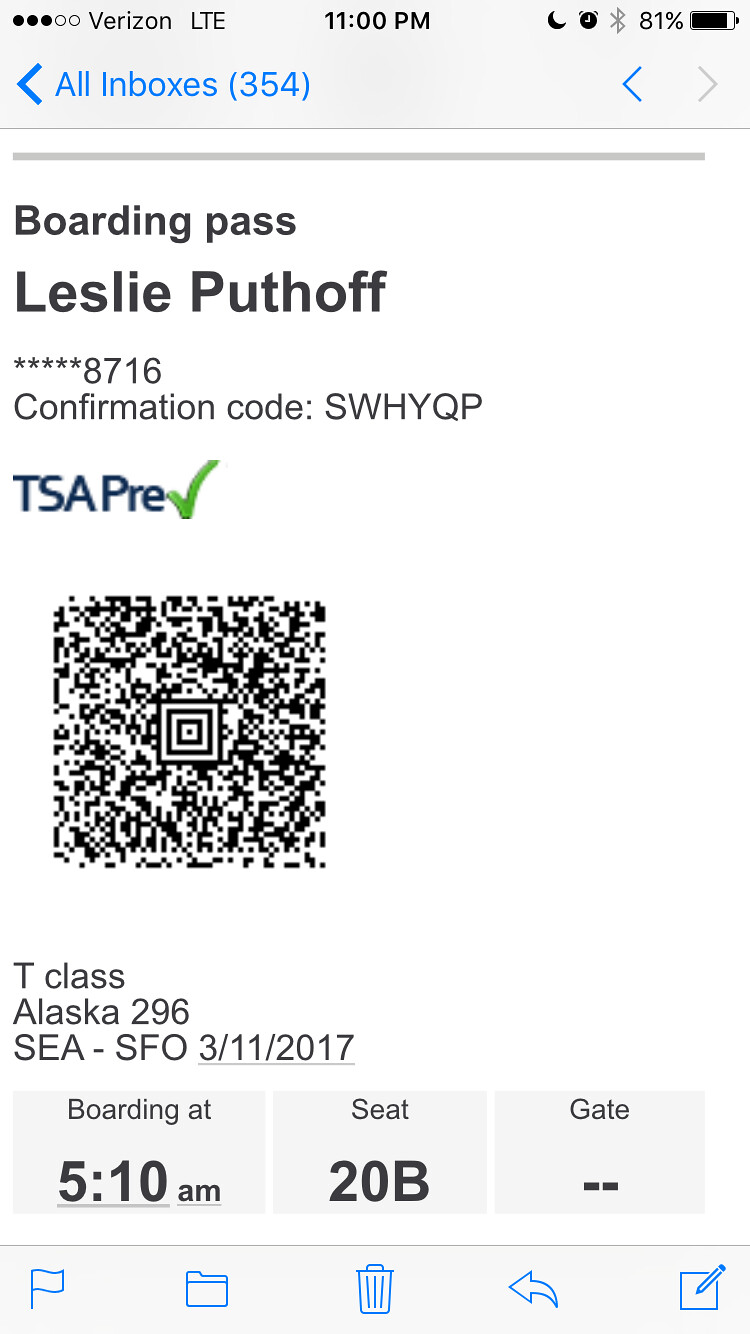The image is a screenshot of a cell phone, indicated by details such as the Verizon LTE signal on the left, the 81% battery level on the right, and the time displayed as 11 p.m. The main content of the screen is an email app showing "All Inboxes" in blue text, with the email displaying a boarding pass for Leslie Puthoff. The boarding pass includes various details in black lettering: the last four digits of her credit card, her confirmation code, and a TSA PreCheck status denoted by a green checkmark. A QR code is present along with flight details, specifying a t-class Alaska Airlines flight 296 from SEA to SFO, departing on 3/11/2017, with boarding at 5:10 a.m., and seat assignment 20B. At the bottom of the email, there are control options labeled as flag, file, delete, share, and write.